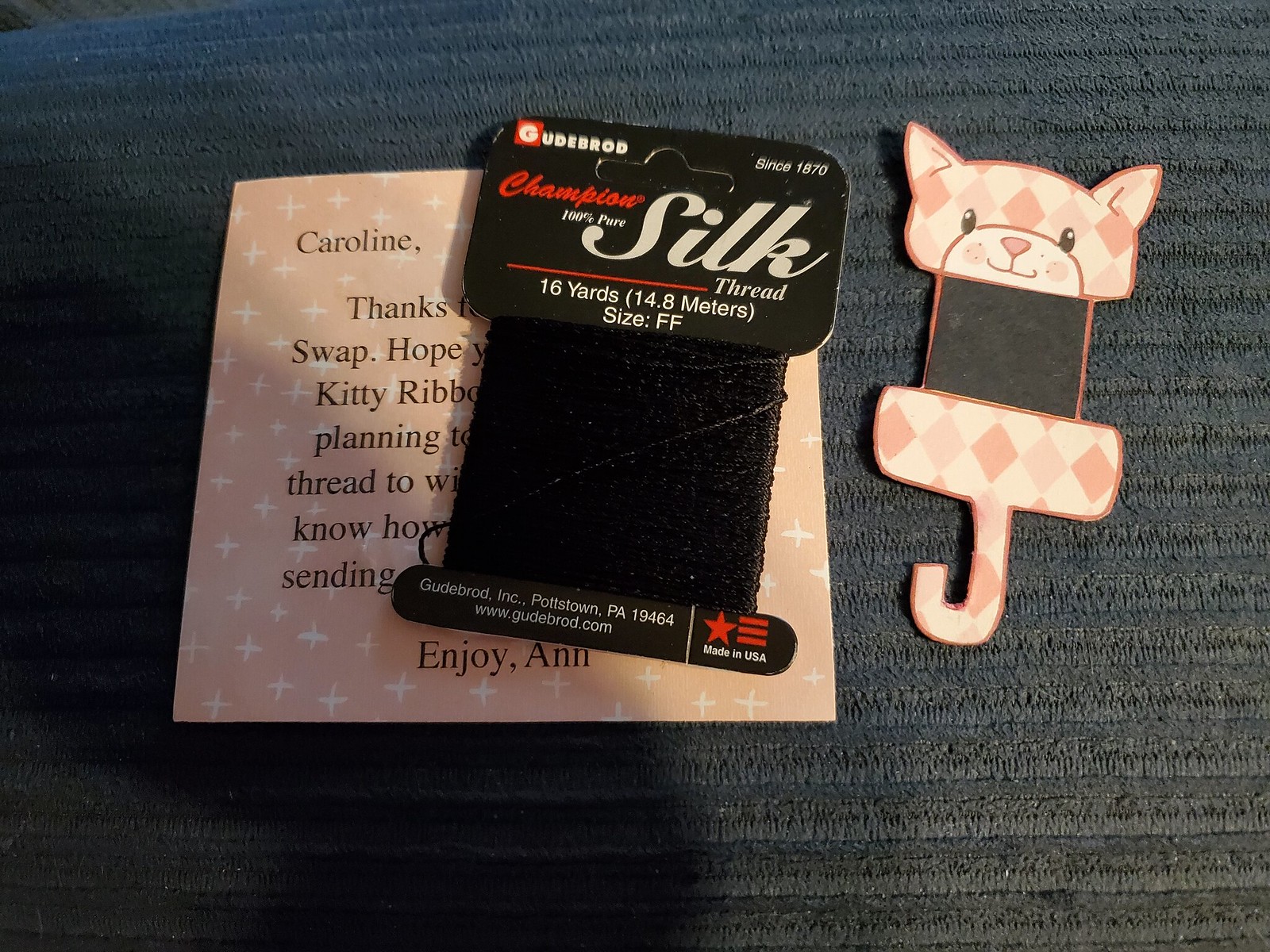This detailed indoor photograph features a centrally placed spool of Champion 100% pure silk thread, wrapped around a cardboard insert. The insert displays a variety of text: "Goodebrod since 1870," "Champion 100% pure silk thread," "16 yards, 14.8 meters," "size FF," and "Goodebrod Inc., Pottstown, PA 19464, Made in USA." The predominantly black insert contrasts with its surroundings. Directly beneath this spool, a partially obscured pink and white note card peeks out, adorned with black text—some visible words include "Caroline," "thanks," and "Anne." To the right of the spool, a cat-shaped hanger similarly wrapped in silk continues the crafty theme, with a cat's head, body, and tail distinctly shaping the object. Overall, the image gives an impression of an arts and crafts setup, possibly in a cozy corner of someone's home, with the scene set against dark fabric or a cushion, bringing focus to the various elements of silk, paper, and feline-themed tools.